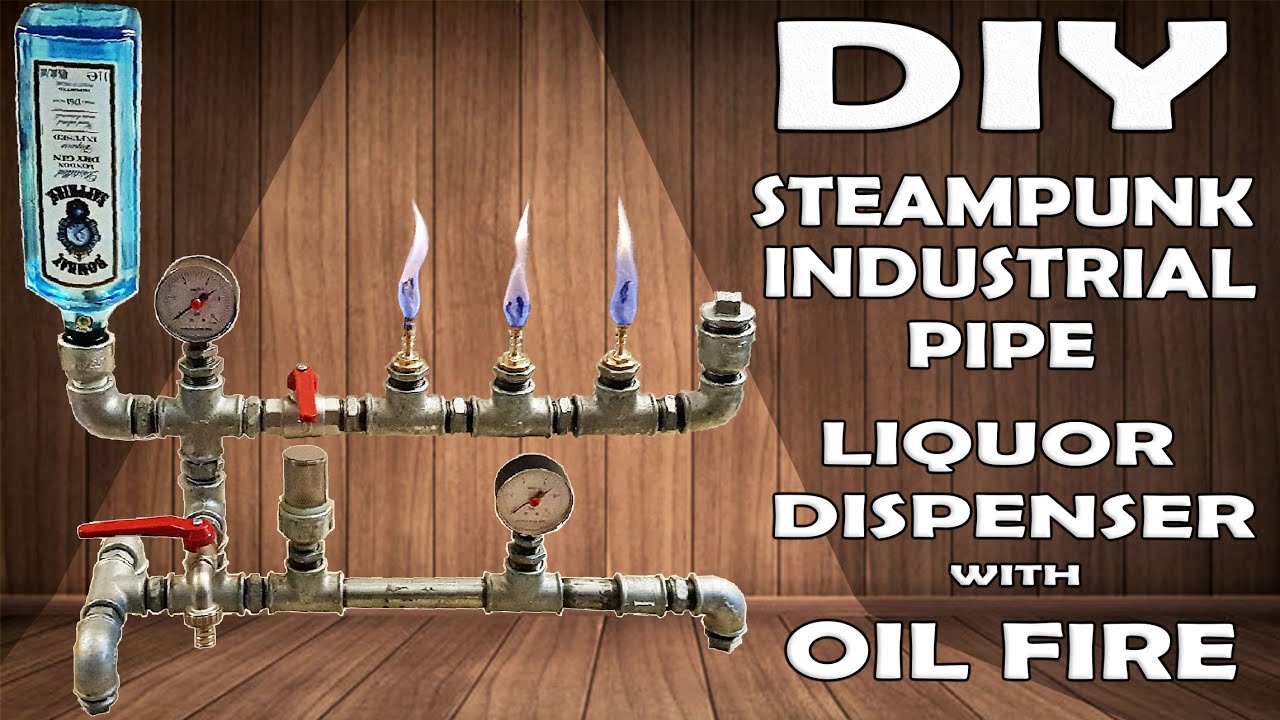The image showcases a detailed illustration of a DIY Steampunk Industrial Pipe Liquor Dispenser with Oil Fire. Set against a background of wooden slats in a brown hue, the graphic features a complex arrangement of pipes. There are two horizontal pipes connected by a vertical pipe, with additional intricate pipework. A blue, inverted liquor bottle feeds into the upper pipe. The upper pipe is equipped with three burners emitting bluish-white flames, lending an industrial feel to the scene. Key components include two meters: one on the lower pipe and one on the central vertical pipe, as well as a distinctive red faucet on the lower pipe. The right side of the image prominently displays text in white capital letters with a thin dark border, detailing the contraption's DIY nature and steampunk aesthetic.